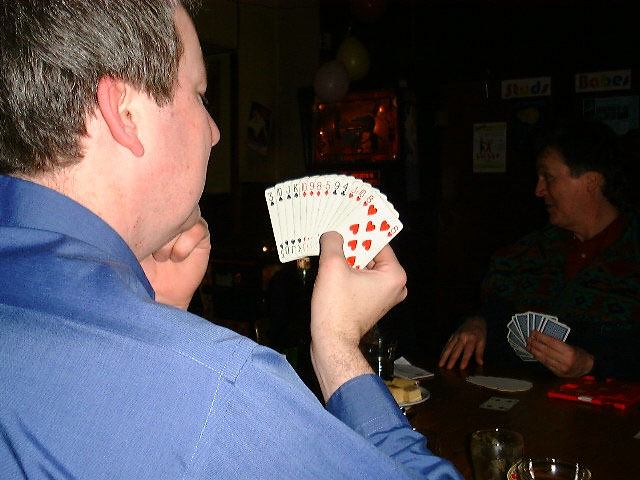In a dimly lit setting resembling a cozy bar or someone's home, a group of people are engaged in an intense card game. The background is dark, partially illuminated by some subtle, dim lights mounted on the wall, adding to the intimate atmosphere. 

At the center of the action is a man, heavily illuminated by a flash that starkly lights up the side of his face and the meticulously arranged cards in his right hand. He appears to be focused, contemplating his next move, with a selection of cards from different suits—hearts, clubs, diamonds, and spades—ordered neatly. Notably, the 8 of hearts is visible at the end of his hand.

This man is wearing a blue long-sleeved shirt, and has short dark hair flecked with hints of gray. Across the table sits another player, clutching cards with blue backs in his left hand. He is turned slightly to the left, likely engaged in conversation with someone not visible in the frame, suggesting that the game involves more participants.

The table between them is cluttered, presumably with drinks and other items, although the flash's illumination makes it difficult to discern specifics. The overall ambiance is one of relaxed camaraderie and strategic concentration, typical of a friendly but serious card game session.